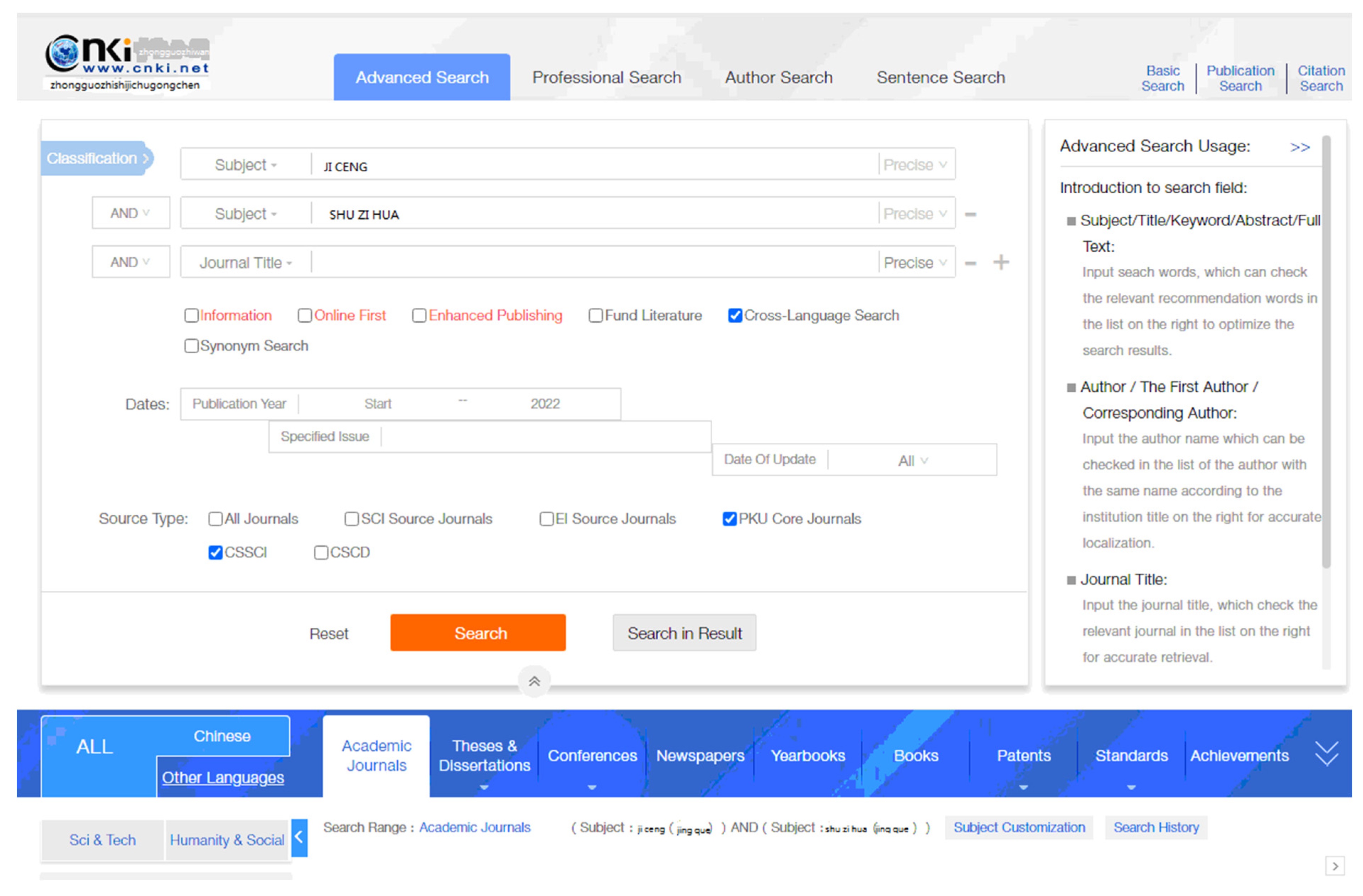A screenshot of a web page is displayed with a low resolution, making the text challenging to read. In the upper left corner, there is a symbol accompanied by the name "ONKI" and the URL "www.onki.net" positioned directly below it. The image showcases several menu options such as "Advanced Search," "Professional Search," "Author Search," "Sentence Search," located to the right of the main text, and "Basic Search," "Publication Search," and "Citation Search."

The page also contains various input boxes for users to fill in, including classifications, subjects, precise search terms, and journal titles. Users can input potentially multiple words in these boxes, but specific terms used in the subject box are unclear. There are also numerous checkboxes for further customization, such as dates and source types. At the bottom of the screen, there are three buttons labeled "Reset Search," "Search," and "Results." Additionally, to the right side of the image, there are further menu options labeled "Advanced Search Usage" and "Description."

Overall, the interface appears to be a detailed search page designed for intricate and precise academic or professional research.